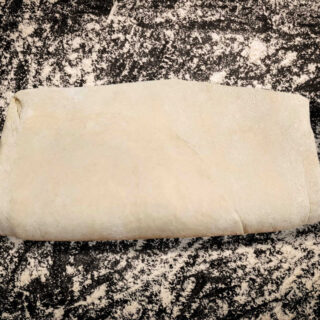The image features a monochromatic background with a streaky, marble-like pattern, reminiscent of a black worktop dusted with flour. Placed centrally in the scene is a rectangular, smooth white object, folded on one side towards the viewer. The object's texture and appearance suggest it is puff pastry, poised and ready on the floured worktop, awaiting the next roll in its preparation process. This setting, rich in texture and implied action, captures a moment of culinary anticipation.